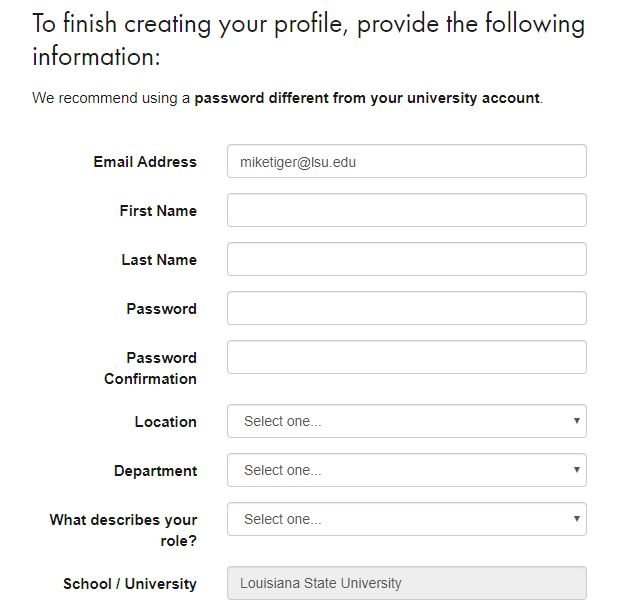The image features a clean, white background with instructions for completing a profile creation process. The top of the image contains the statement: "To finish creating your profile, provide the following information." Below this are fields for inputting an email address, which is pre-populated with "miketiger@lsu.edu," as well as boxes for entering a first name, last name, password, and password confirmation. There is a prompt recommending the use of a password different from your university account password.

Further down, there are drop-down menus for selecting a location, department, and role description, each featuring a "Select one" option alongside a down arrow indicating more choices. Lastly, there is a field for specifying the school or university, which is filled in with "Louisiana State University (LSU)." The overall message emphasizes the need to complete this form by entering the necessary personal information to finalize the profile creation.